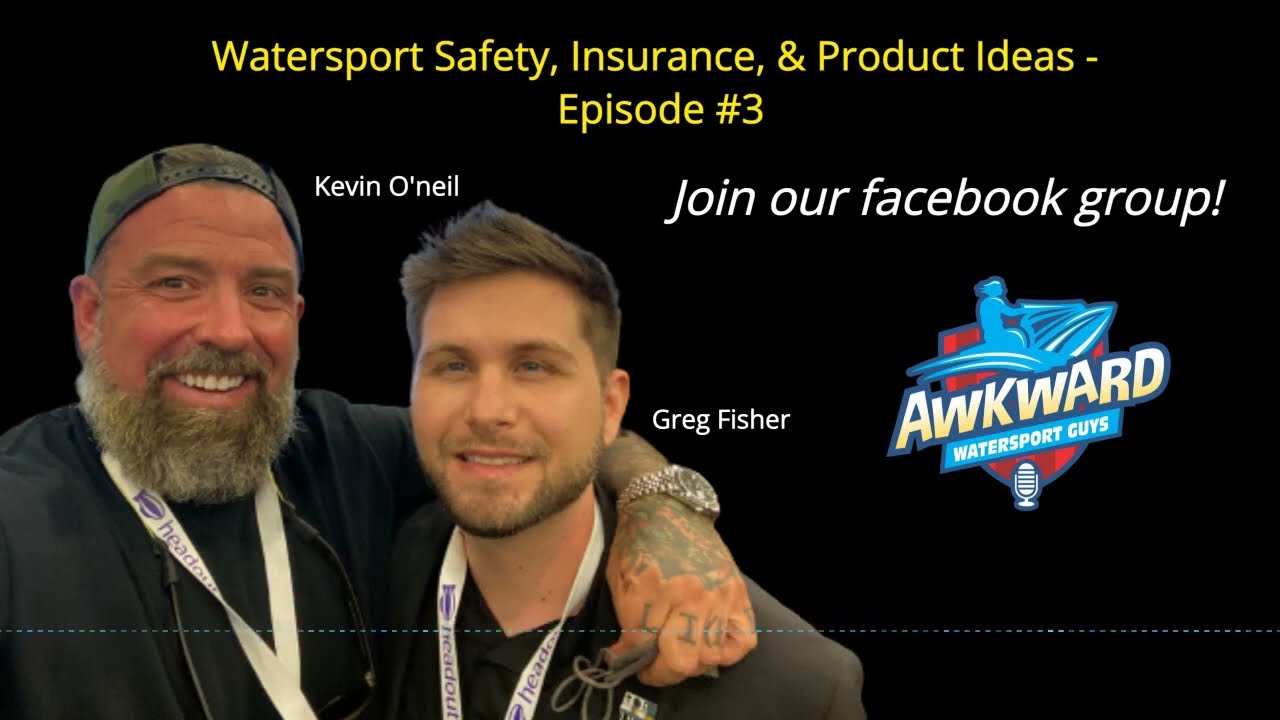The image is the thumbnail for a YouTube video for the show "Awkward Water Sport Guys," Episode 3, titled "Water Sports Safety Insurance and Product Ideas." At the top, it reads, "Water Sports Safety Insurance and Product Ideas, Episode Number 3," with a call to action underneath that says, "Join our Facebook Group." Below this, there is a brand logo featuring an illustration of a person on a jet ski and an icon of a microphone. In the center of the image, two men are featured. On the left is Kevin O'Neill, wearing a backwards green baseball cap and a black shirt, with a fairly long, black and white beard. He has his arm around Greg Fisher, who appears younger with short brown hair and a shorter beard. Both men are smiling, have white lanyards around their necks, and are dressed in black shirts.